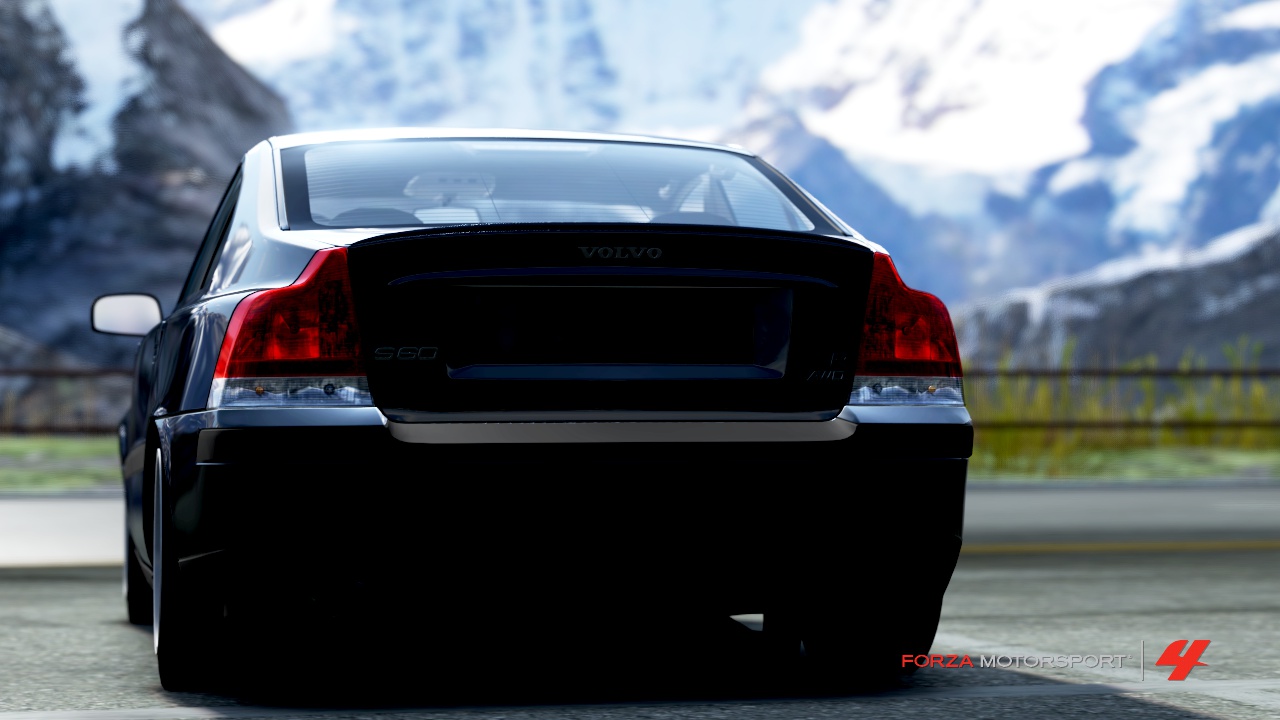This detailed photo captures the rear of a dark blue Volvo S60, prominently showcasing the Volvo logo at the top center of the trunk lid, with the S60 badge on the bottom left and an all-wheel drive badge on the bottom right. The iconic red and white tail lights add to the vehicle's distinct look. The car is parked in what appears to be a parking lot, close to a sidewalk and a barrier. Behind the barrier, there's vegetation and grass, with snow-covered mountains, possibly the Swiss Alps, visible in the bright daytime sky. This image, with the Forza Motorsport 4 logo featured in the bottom right corner—'Forza' in red and 'Motorsport' in white—suggests that it might be a highly detailed 3D rendering or a still from the Forza Motorsport video game, rather than a photograph taken in a real setting.